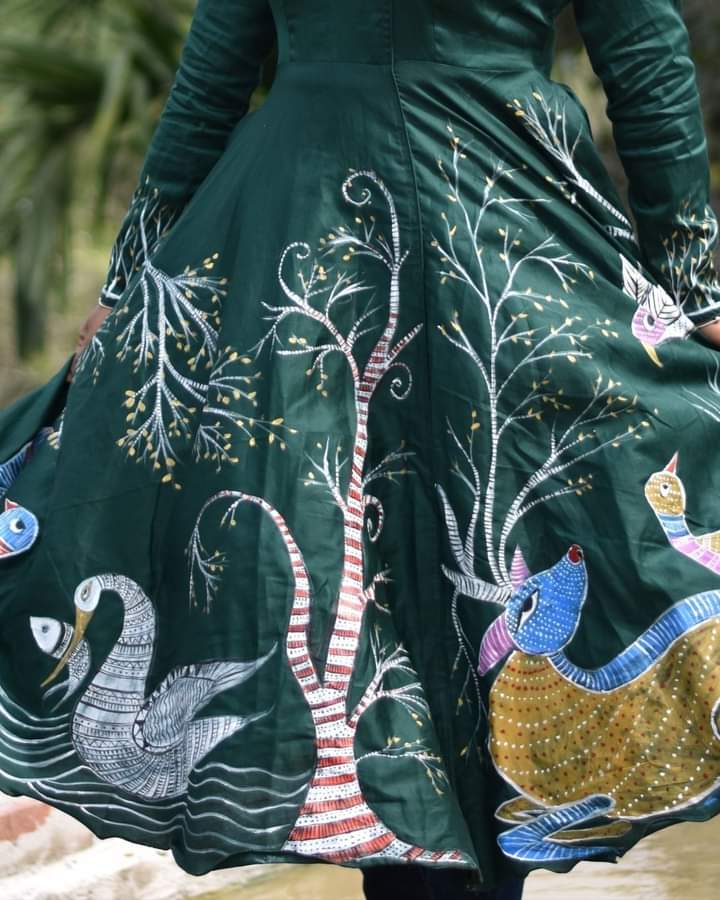This photograph features a striking, emerald-green dress, captured from the midsection down, worn by a woman standing outdoors. The image is taken vertically, encompassing the dress from her waist to her knees. The dress fabric is adorned with intricate, vibrant embroidery that brings a whimsical, almost fantastical scene to life. 

The dress has long sleeves, extending to the wrists, with cuffs embroidered in a green and white pattern reminiscent of flames. The skirt, held outward by the woman’s hands, reveals the elaborate design against the dark green background. On the left side of the dress, a majestic white swan is depicted with its wings spread and a fish held in its yellow beak, surrounded by embroidered water ripples and additional fish. Moving upward, a red-and-white-striped tree with curly branches grows from the bottom of the skirt to the midriff, adding to the enchanting scene.

To the right, a reclining golden goat with red and white dots features prominently, adorned with a blue face, red nose, and red-striped ears. Further up, more white branches with buds expand outward and upward. The overall impression evokes a sense of charming wonder, blending elements of classical art with a magical, almost Alice in Wonderland-like aesthetic.

In the blurred background, we discern hints of greenery and possibly water, suggesting the woman might be standing in a natural outdoor setting, enhancing the organic feel of the dress’s design. The dress and its detailed embroidery, set against the emerald green fabric, form a visually captivating and richly detailed piece of wearable art.